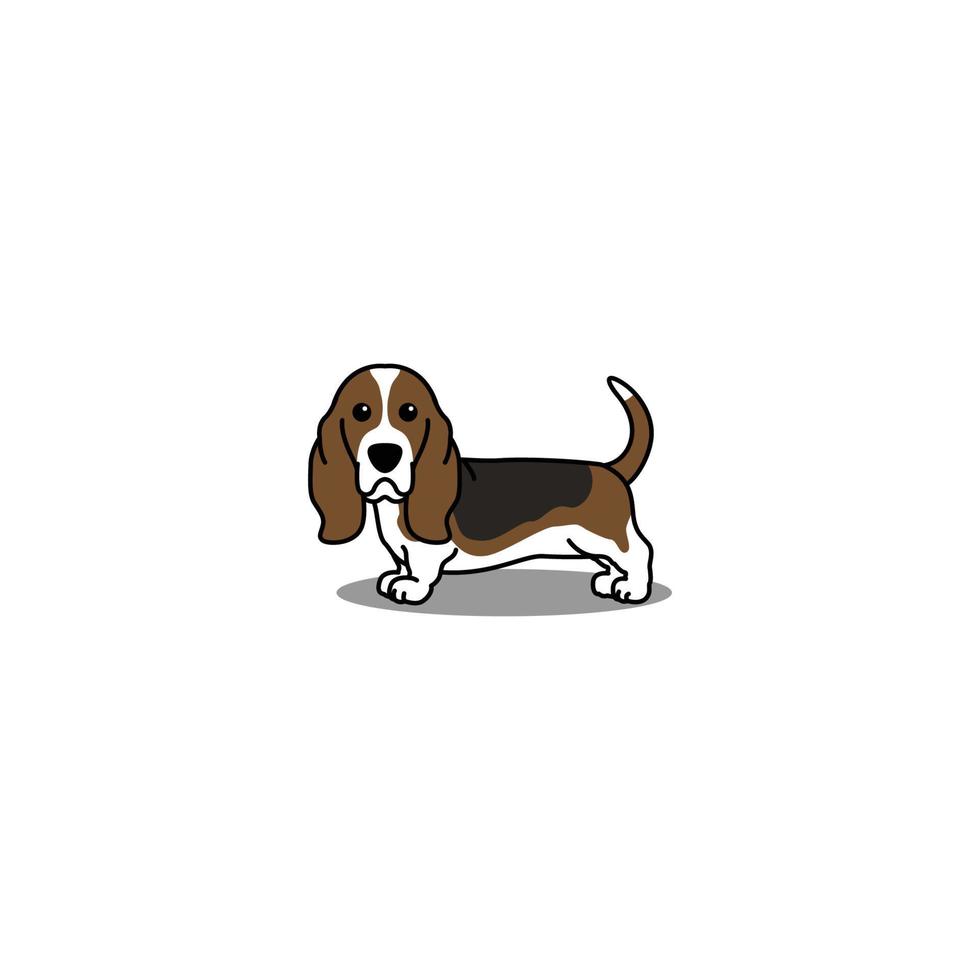The image depicts a digital cartoon line art drawing of a basset hound. The background is completely white, highlighting the simplistic yet detailed design of the dog. The basset hound is shown with a long, elongated body and very short, stubby legs, making its stomach hang low to the ground. The dog’s most striking features include its long, droopy ears and a distinct, largely brown face with a black nose and expressive, beady black eyes that appear teary.

The dog's color palette is a mix of brown, white, and hints of black. The ears and area around the eyes are brown, while a white stripe runs down the center of its face and around its mouth. The dog’s underbelly, chest, and the tip of its tail are also white, whereas its back comprises various shades of brown, from dark to lighter tones. The tail, pointing upwards, is predominantly lighter brown with a white tip.

The dog is positioned as if looking directly at the viewer, with its head slightly turned to present a clearer view of its facial features. The image also includes a subtle, gray oval shadow beneath the dog, giving it an anchored and three-dimensional appearance despite the overall simplicity of the graphic.